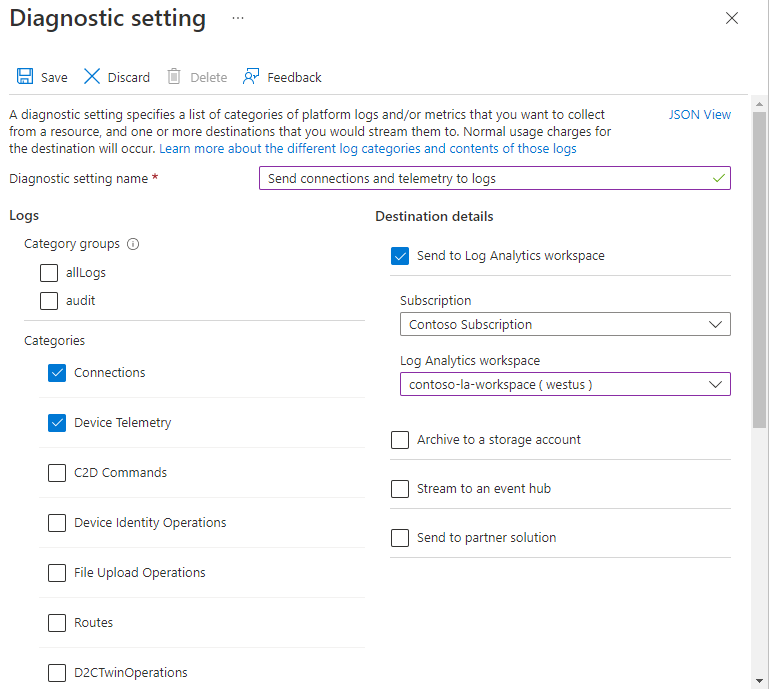**Detailed Caption: Screenshot of Diagnostic Settings Panel**

The screenshot captures a detailed view of the Diagnostic Settings panel. Positioned in the top left corner, the title 'Diagnostic settings' is highlighted in large black font. On the top right, there is a close button marked with an 'X'. Alongside, icons for various functionalities are neatly arranged: a blue floppy disk labeled 'Save', a blue 'X' for 'Discard', a grayed-out trash can, a grayed-out 'Delete', and an icon featuring a person within a speech bubble which is meant for 'Feedback'.

The panel describes that diagnostic settings specify all the categories of platform logs and/or metrics to be collected from a resource, and the destinations to which they are streamed. It notes that normal usage charges for the destination will apply. Below this, a blue hyperlink invites users to "Learn more about the different log categories and contents of those logs."

Beneath this, there is an input field for naming the diagnostic setting, currently filled out with "send connections to telemetry and telemetry to logs." The settings for logs allow various options like checking all logs and auditing. The option to 'Send to log analytics workspace' is selected, grouped under 'Category Groups'.

Further down, there are checkboxes for different categories. On the left side, there are seven categories including 'Connections' and 'Device telemetry', which are selected. The others, namely 'C to D commands', 'Device identity operations', 'File upload operations', 'Routes', and 'D to C twin operations', are not selected. On the right side, three more categories remain unchecked: 'Archived to a storage account', 'Streamed to an event hub', and 'Sent to a partner solution'.

Overlaying dropdown menus and options add further detail to the interface. The section 'Subscription details' lists 'Contoso subscription' and 'Contoso LA Workspace Westis', emphasizing the context of usage.